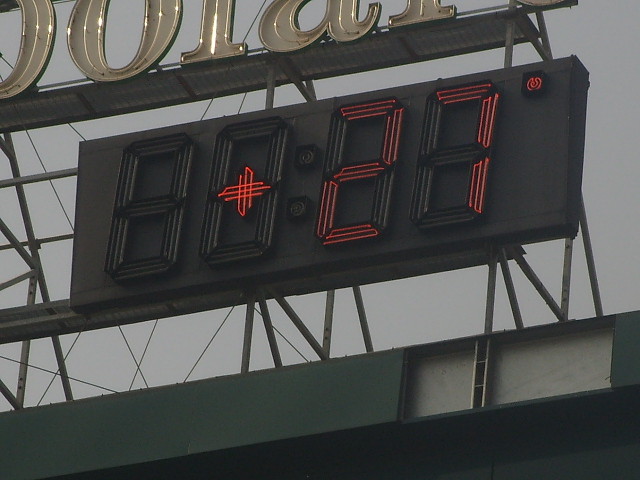A large, digital temperature display is mounted prominently atop a building, reminiscent of the way lights are installed on stadium roofs. The roofline, which appears in a muted gray-green hue, stands out against a dull gray sky in the background. The temperature readout is enclosed in a substantial black square, highlighting a red, digital "+27 degrees" with neon lighting—a brighter and more prominent plus sign compared to the "27." Positioned above the temperature display, shiny gold lettering—likely indicating a sponsor—is partially visible, though the entirety of the text is cut off by the edges of the photograph.